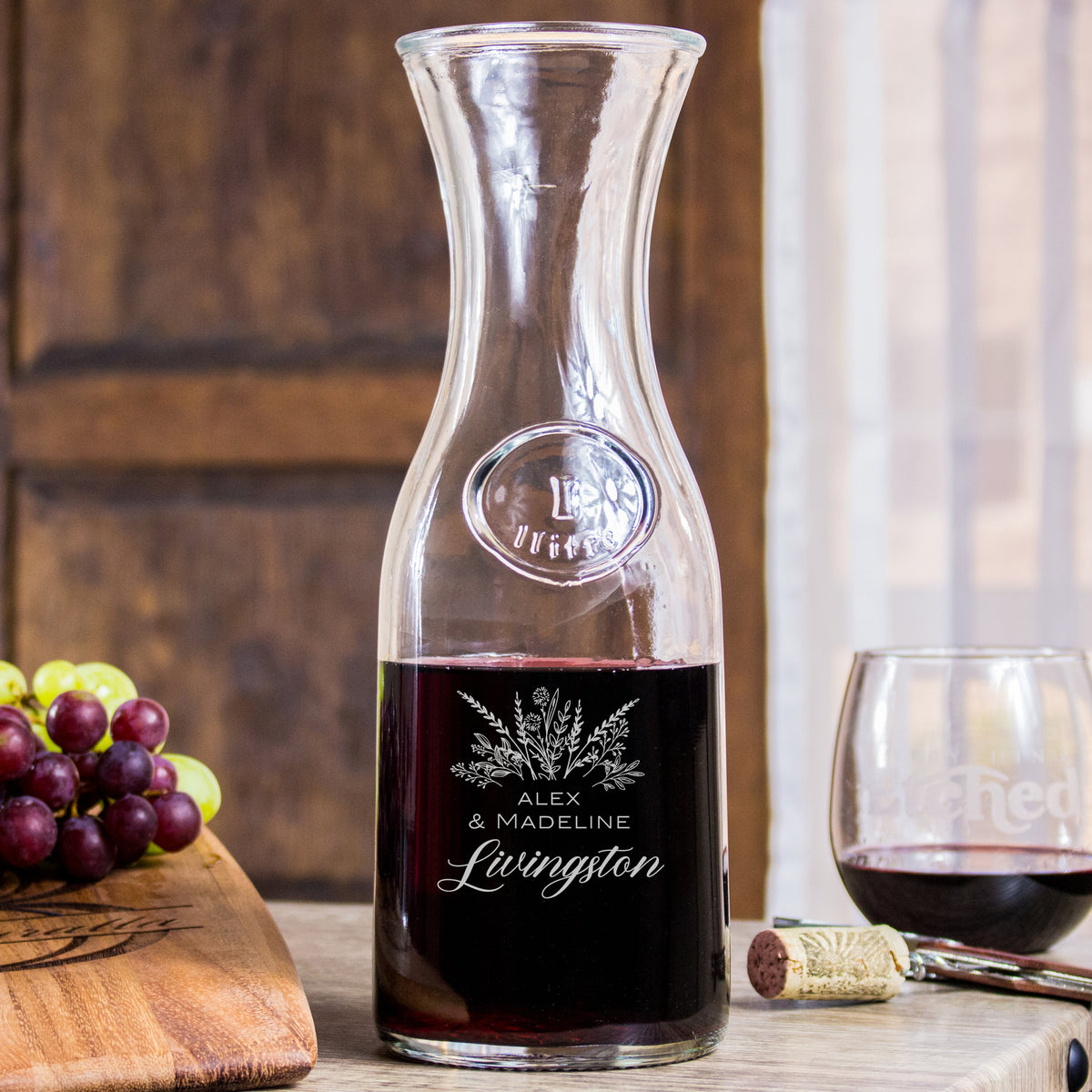The photograph captures a beautifully arranged indoor setting with a distinctly warm and inviting ambiance. The backdrop features a medium-toned brown wall with subtle black streaks, complemented by a sheer curtain through which vertical white blinds are visible, creating a soft, diffused lighting effect. Central to the image is a light blonde wooden table, characterized by darker streaks that add texture and character.

On this table sits a prominent glass wine decanter, intricately shaped with a squared body that curves at the neck. The decanter is adorned with delicate etchings of plant life, including wheat, leaves, and blossoms, giving it an artistic flair. In an oval at the base, the names "Alex and Madeline" are printed, while "Livingston" is elegantly scripted below. The decanter is filled halfway with a dark red wine.

To the right of the decanter, a cork lies next to a stemless wine glass, which is etched with the word "etched" and is filled a third of the way with the same rich red wine. In front of the glass, a light tan cork with an olive green sun decoration is placed alongside a metal bottle opener.

To the left of the decanter, a wooden cutting board holds two clusters of grapes—one green and one purple, adding a touch of vibrant color to the setting. The overall composition, with its blend of rustic and elegant elements, evokes a scene of relaxed sophistication and timeless charm.